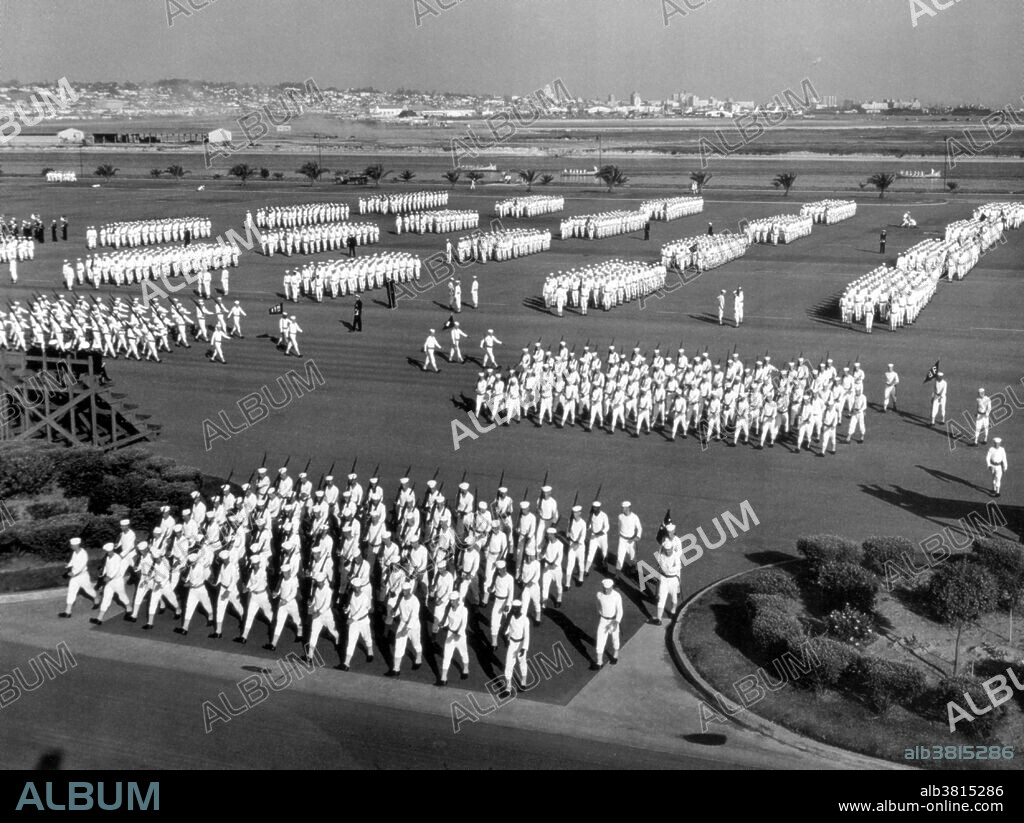This black-and-white image presents a wide military parade or training session, taking place on a vast, flat airfield. The soldiers are meticulously arranged in horizontal and vertical formations, dressed uniformly in white from their hats to their shoes. Numerous groups are visible, each consisting of about four to five lines of men, with distinct spaces separating them.

Towards the top of the image, the horizon reveals city buildings and a visible sky, setting an urban backdrop. In the foreground, closer to the camera, two groups of soldiers appear to be marching directly towards the viewer, while additional groups move from left to right across the field. On the left, there's a set of bleachers indicating a stadium, and to the front right, a small garden with dark gray trees and bushes adds contrast. Some soldiers, particularly those in the bottom center, are carrying guns.

A light white watermark reading "album" is stamped prominently over the image, and a black border at the bottom left contains the same text in teal along with the identifier "ALB 3815286" and the URL "www.album-online.com."